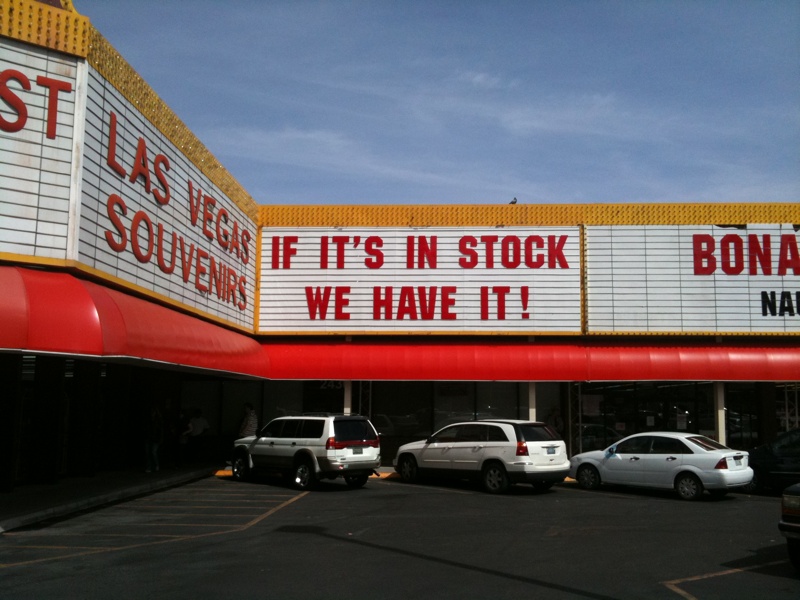The image showcases the exterior of a retail store named "Las Vegas Souvenirs" set against a clear blue sky dotted with a few cirrus clouds. The store's name is prominently displayed on a marquee board reminiscent of a theater's, with a gold border framing the red letters that spell out "Las Vegas Souvenirs." Adjacent to this, another marquee board reads, "If it's in stock, we have it." Below these boards, a red awning stretches across the storefront. The lower part of the image reveals a parking lot where three white vehicles are parked side by side: the first two appear to be sport utility vehicles, while the third is a sedan. The image focuses closely on the building, limiting the view of the parking area to just these three cars.